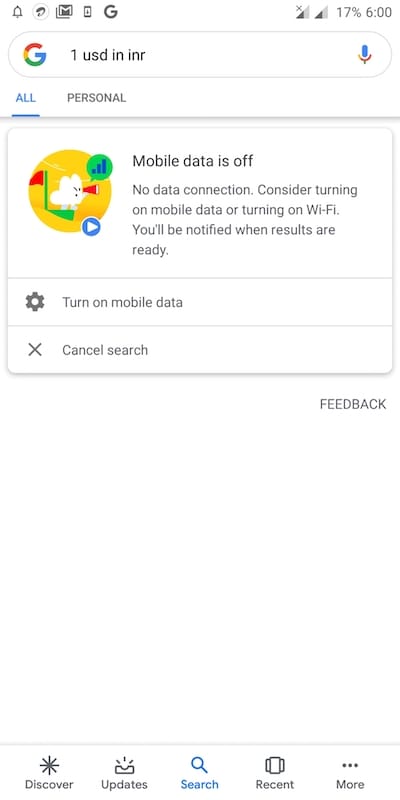The screenshot displays a mobile device interface with various notification icons on the status bar. Starting from the left, there is a bell icon indicating a notification alert, followed by an unidentified icon. This is succeeded by a Gmail notification, a phone notification, and a Google notification. The Google app is actively open, showing a search query for "1 USD in INR." However, a message indicates that mobile data is turned off, leading to no data connection. The user is prompted to either turn on mobile data or connect to WiFi, with options to enable mobile data or cancel the search.

At the bottom of the screen, there are navigation options labeled Discover, Update, Search, Recent, and More. The top of the screen shows an 'X' next to the network signal icon, indicating no signal, a battery icon displaying 17% remaining charge, and the current time set at 6:00.